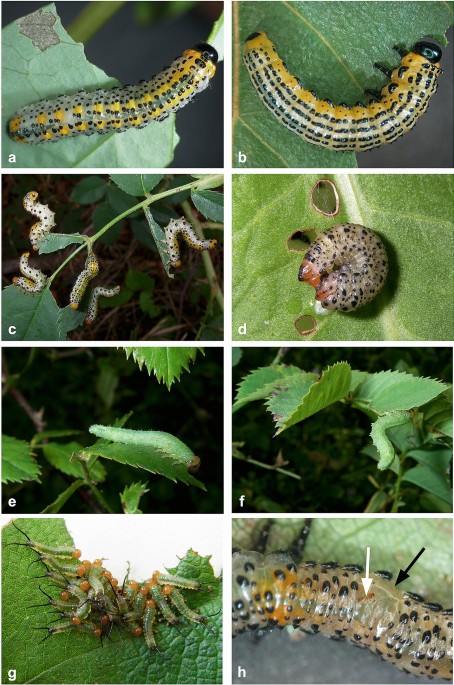The image is a vertical rectangle composed of eight square photographs of caterpillars, arranged in two columns and four rows. Each photograph is labeled with a letter (A–H) in the bottom left corner. 

Starting from the top-left, Picture A shows a yellow and black caterpillar with a gray body and black spots, situated on a green leaf. In Picture B, the same caterpillar appears in a different position, with black and white markings and tan lines along its top, featuring a black head. Moving down to Picture C, various caterpillars are seen hanging from a branch, each with white bottoms and sharp, pointy black feet. Picture D displays a gray caterpillar with black spots, curled up into a ball on a leaf with visible holes.

In the right column, Picture E shows a green caterpillar resting on a leaf, camouflaged against the green background. Picture F portrays another green caterpillar hanging from a leaf, similarly blending into its surroundings. Moving down to Picture G, the image captures a half-eaten leaf with multiple smaller caterpillars hanging off of it. The final image, Picture H, is a close-up of a caterpillar with a translucent tan body, black spots, and a yellow patch, featuring white and black arrows pointing to specific areas on its body.